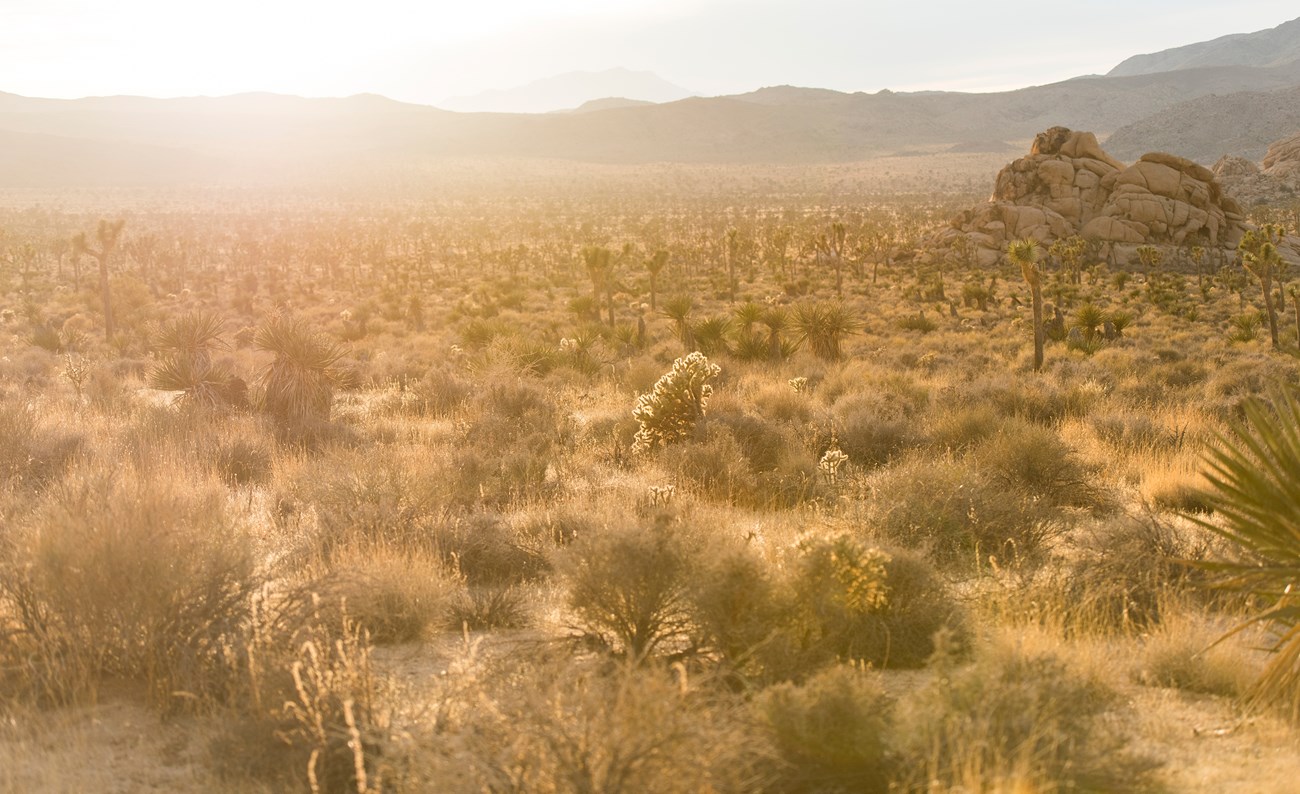This dynamic photograph captures a vivid desert landscape that is predominantly brown, highlighted with occasional green and black grasses. In the middle of the image, a striking plant with green leaves that transition to white or brown at the tips stands out. Scattered throughout the scene are various desert plants, including thin-leaved bushes and several types of cacti, adding diversity to the arid terrain. The ground itself is a patchwork of brown dirt and sparse sand, typical of a desert environment. To the right, a distinctive rock formation rises about 10-15 feet, creating a small hill devoid of foliage. In the distance, a rugged mountain range stretches across the horizon from left to right, set beneath a clear blue sky. The photograph is distinctly bright, indicating it was taken during the day, with sunlight illuminating the path, particularly in the top left corner. This interplay of light enhances the landscape's textures and tones, creating a captivating and detailed depiction of a desert scene.